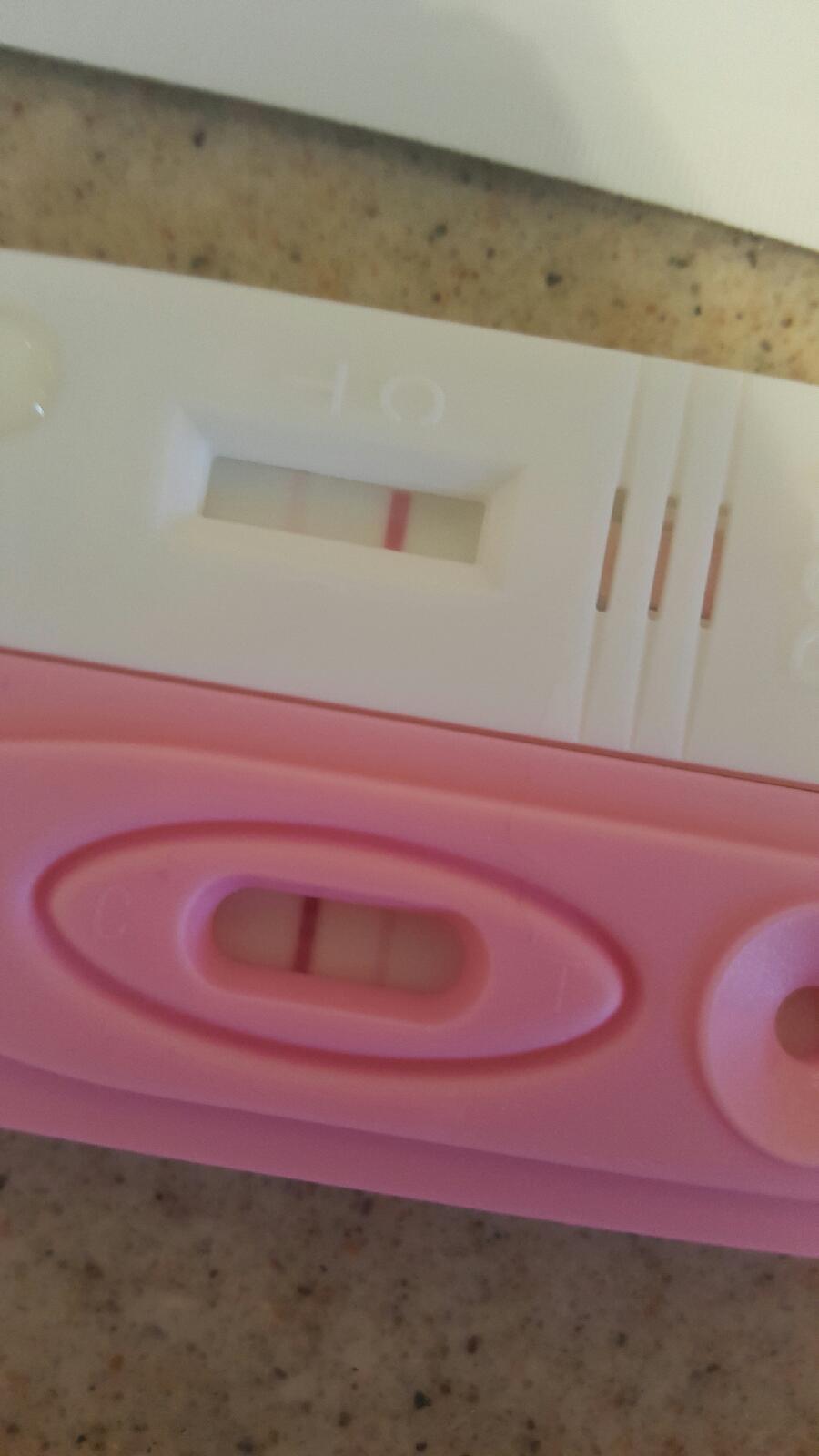This color image captures two plastic rectangular devices, indicative of pregnancy tests, positioned one atop the other at a slight horizontal angle. They rest on a white countertop marred with dark marks and blemishes, suggesting a well-used surface. The bottom device, constructed from pink plastic, features a rectangular window with rounded corners, displaying two red lines indicative of the test's result. The upper device, made of white plastic, mirrors the pink device in shape and function but lacks rounded edges and showcases a clear rectangular window. Both devices serve the same purpose: detecting pregnancy through the analysis of urine.